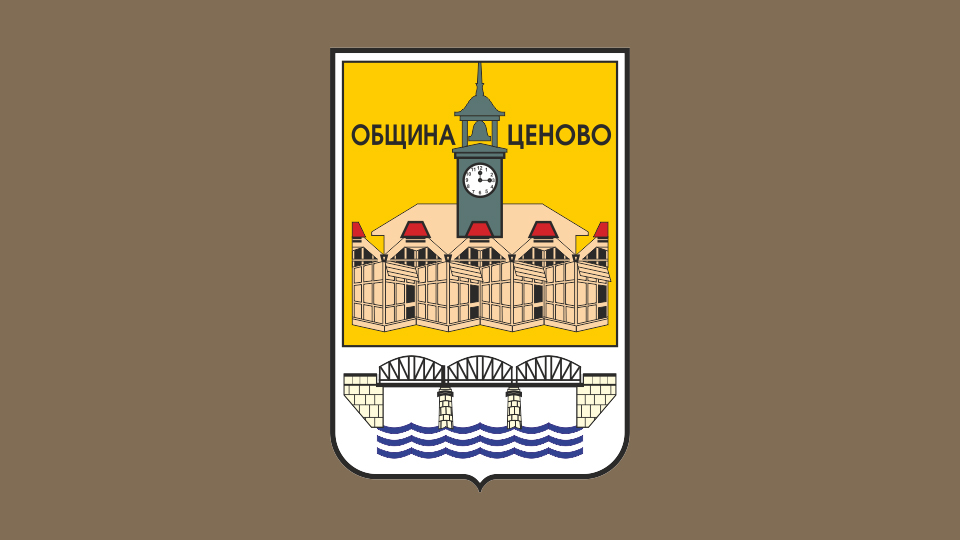This image depicts a computer-generated seal, possibly representing a municipality or government body, set against a light brown background. The seal is shield-shaped with straight upper sides and rounded lower corners, culminating in a small curved spike at the bottom center. The outer border of the shield is solid white.

Inside the shield, a prominent yellow square with a black border contains a detailed illustration of a clock tower, framed by two Cyrillic words. The clock features black hands and numbers on a white face, housed within a dark gray structure topped by a dark gray bell, and flanked by beige walls with red caps.

Below the yellow square, a depiction of a bridge arches over wavy lines, suggesting a body of water. This careful composition blends elements that may symbolize the region's landmarks or historical attributes.